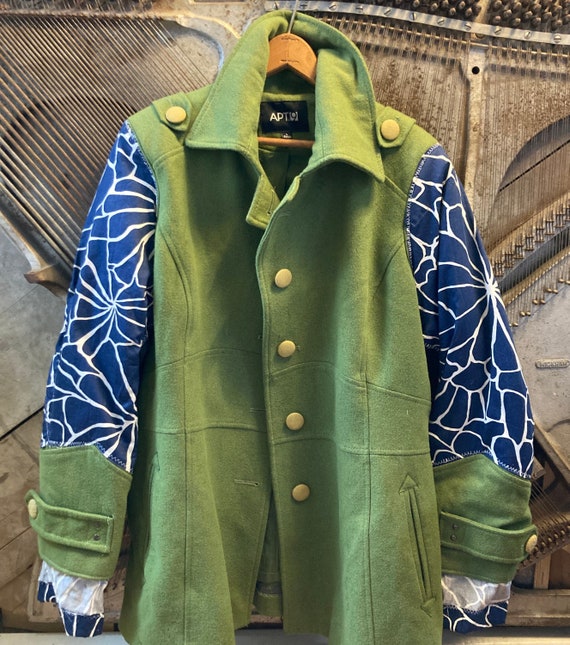This indoor photograph showcases an Apt. 9 vest-style jacket, designed for product advertisement. The jacket, hanging on a wooden hanger, features a predominant suede-like green fabric, described as an olive green. The main body of the garment buttons down the front with distinct pale yellow buttons, complemented by similar buttons on the shoulders and cuffs. The jacket's sleeves add a contrasting visual element with a blue fabric adorned with large white floral prints, which extends from the shoulder to the wrist. The cuffs, crafted from the same green suede material, are adjustable with buttons. Additionally, the jacket includes slit-style pockets on the sides. The entire setup is positioned in front of a backdrop that resembles the interior of an old, rusted string instrument, perhaps a harp, creating a visually intriguing and somewhat industrial background for the product.